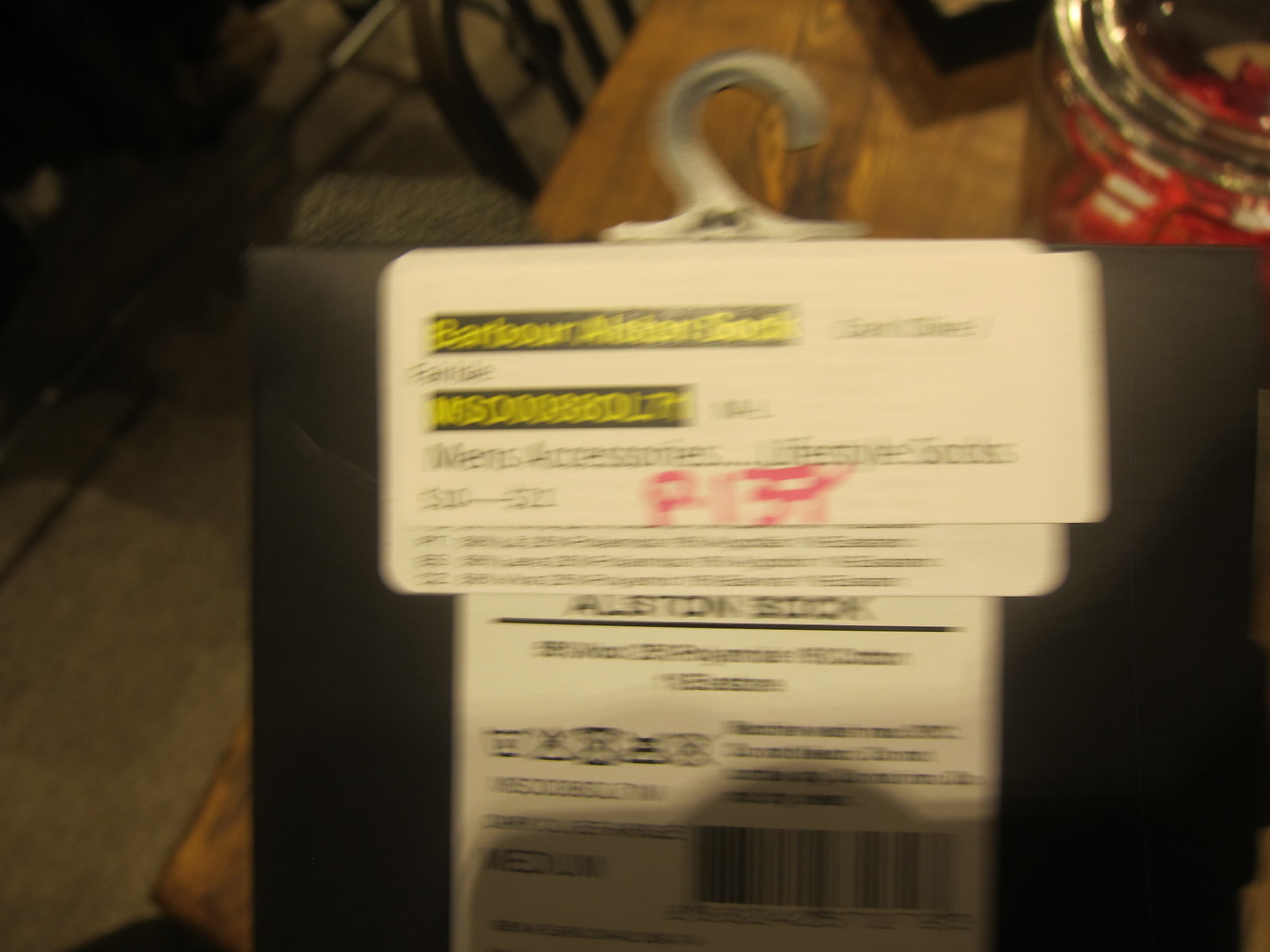This is a photograph of a barber item, most likely boxed and still in the shop, as it is attached to a hanger. The packaging is predominantly black with a large, bold white label on top. The word "Barber" is prominently displayed in yellow letters against a black background. Below this, additional text in the same font and color mentions "Men's Accessories" and "Lifestyle." There is a model or serial number, "B139," written in red, followed by the word "Allerton." The label appears to be layered with multiple tags, one of which includes a barcode and some Chinese writing at the bottom. The size is identified as medium. The image is somewhat blurry, shot under natural lighting, making some text difficult to read.